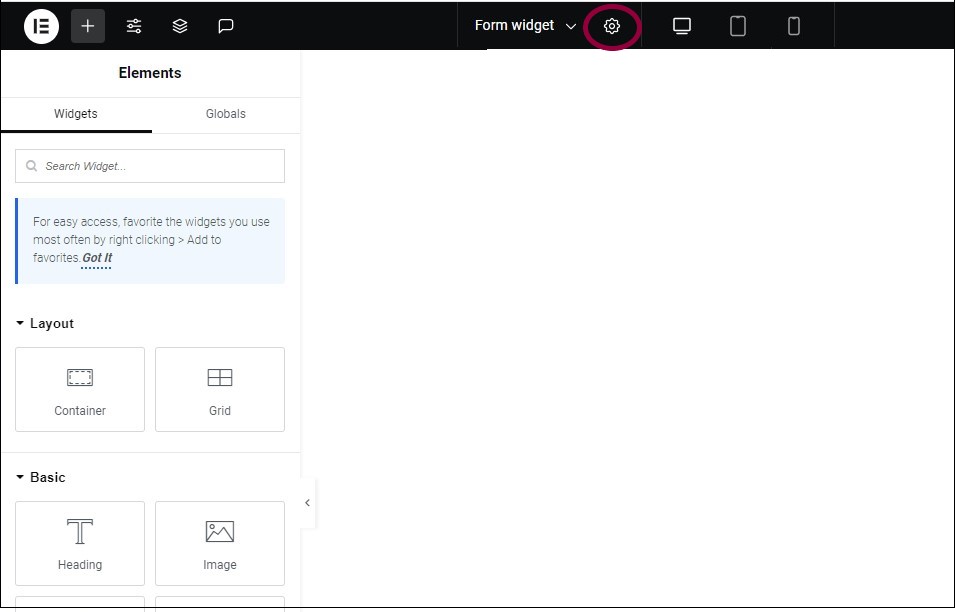The photo captures a dashboard interface for widget settings, presenting a detailed navigational layout. At the top of the image, a horizontal black bar extends from left to right, adorned with white icons. From left to right, the icons consist of a round symbol with a white circle containing a black 'E' in the center, followed by a plus sign, a settings icon, and two additional icons.

Towards the center-right of the screen, there is a form widget with a drop-down arrow option, adjacent to a gear icon—which typically signifies settings. Continuing to the right, there are symbols representing different device types: a PC, a tablet, and a cell phone, suggesting responsive design options.

The left section of the interface features a menu currently set to the widgets tab. This menu allows users to choose various layout options and includes a basic section, indicative of a website creation or customization page. The overall layout and iconography suggest a user-friendly environment designed for managing and configuring widgets on different devices.